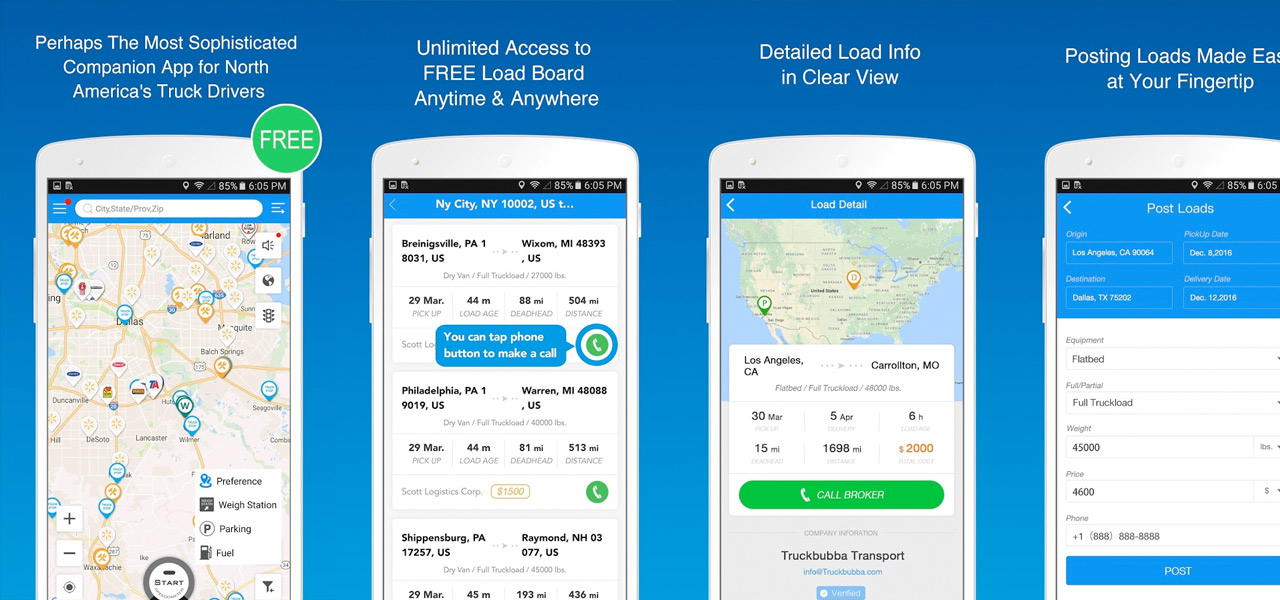The image features a set of identical white-framed cell phones displayed against a gradient blue background that transitions from a dark blue at the top to a lighter blue at the bottom. Each phone showcases different truck-related map and data information.

At the top of the image, above the phones, there's white text providing descriptions and additional information relevant to North American truck drivers. The first phone on the far left is marked with a green circle labeled "Free" in white font. Above it, a caption reads: "Perhaps the most sophisticated companion app for North American truck drivers." The phone's screen displays a map with various icons related to weight stations, parking, and fuel options.

Moving rightward, the next phone offers "Unlimited access to free load board, anytime and anywhere." The screen suggests functionalities such as tapping a phone button to make calls, and displays distances and locations pertinent to trucking logistics.

The third phone presents "Detailed load info in clear view," featuring a map of the United States with detailed information about a specific load: from Los Angeles, California to Carrollton, Missouri, specifying it as a flatbed full truckload of 4,800 pounds with a note to "call broker."

The final phone on the right highlights "Posting loads made easy at your fingertips." The phone's display includes various fields for entering destination, equipment type, partial load details, weight, price, and contact phone numbers.

Each phone is designed with a larger button on the left side and a smaller button on the upper right side, providing a consistent interface across all devices.